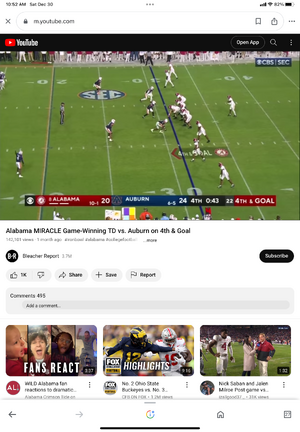A detailed image depicts a smartphone displaying a live football game through a YouTube webpage. The overall layout and proportions suggest the content is being viewed on a mobile device. The top of the screen indicates that the current time is around 10 a.m., and the battery indicator shows a full charge, estimated to be around 80-90%.

Prominently visible is the game between Auburn and Alabama, with the scoreboard reflecting Auburn leading 24 to Alabama's 20 in the fourth quarter during a critical fourth-and-goal situation. The title of the video highlights a dramatic moment: "Alabama Miracle Game Winning TD vs Auburn on 4th and Goal," uploaded by Bleacher Report.

Below the video player, a blue "Subscribe" button invites viewers to subscribe to the channel. There's a visible comments section with a count of 495 comments and an area suggesting users add their own comments.

Thumbnail previews of three additional YouTube videos are also displayed. One thumbnail highlights fans reacting to game highlights, a video provided by Fox. On the right-hand side, another thumbnail shows someone speaking with the coach, but the details are too small to decipher clearly.